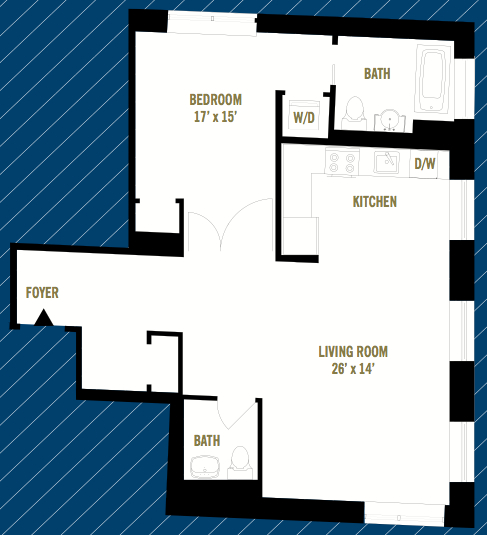The image depicts a simplified blueprint of a house, set against a blue background with white pinstripes running diagonally from the bottom left to the top right. The blueprint is presented on white paper, highlighted by an organically shaped black cut-out that frames the design, emphasizing the empty spaces surrounding it.

Starting from the left, the layout features a centrally located rectangular section labeled "Foyer," which seamlessly connects to a square area at the bottom. Extending downwards at a right angle from the foyer, the blueprint continues towards the right with another right angle, leading to a section marked "Bath." The layout is organized in a series of interconnected squares around the periphery.

In the top left corner, there's a room labeled "Bedroom" with dimensions of 17 by 15 feet, and it includes an area for a washer and dryer. Directly beneath this bedroom, there's an attached bathroom. At the center of the blueprint, an open-plan kitchen is indicated, complete with a dishwasher, which flows into a spacious living room measuring 26 by 14 feet. Adjacent to the left side of the living room and slightly downward, there's a small bathroom positioned before the foyer.

The blueprint includes fine details such as the placement of doors, windows, and major appliances, clearly marked with small lines.